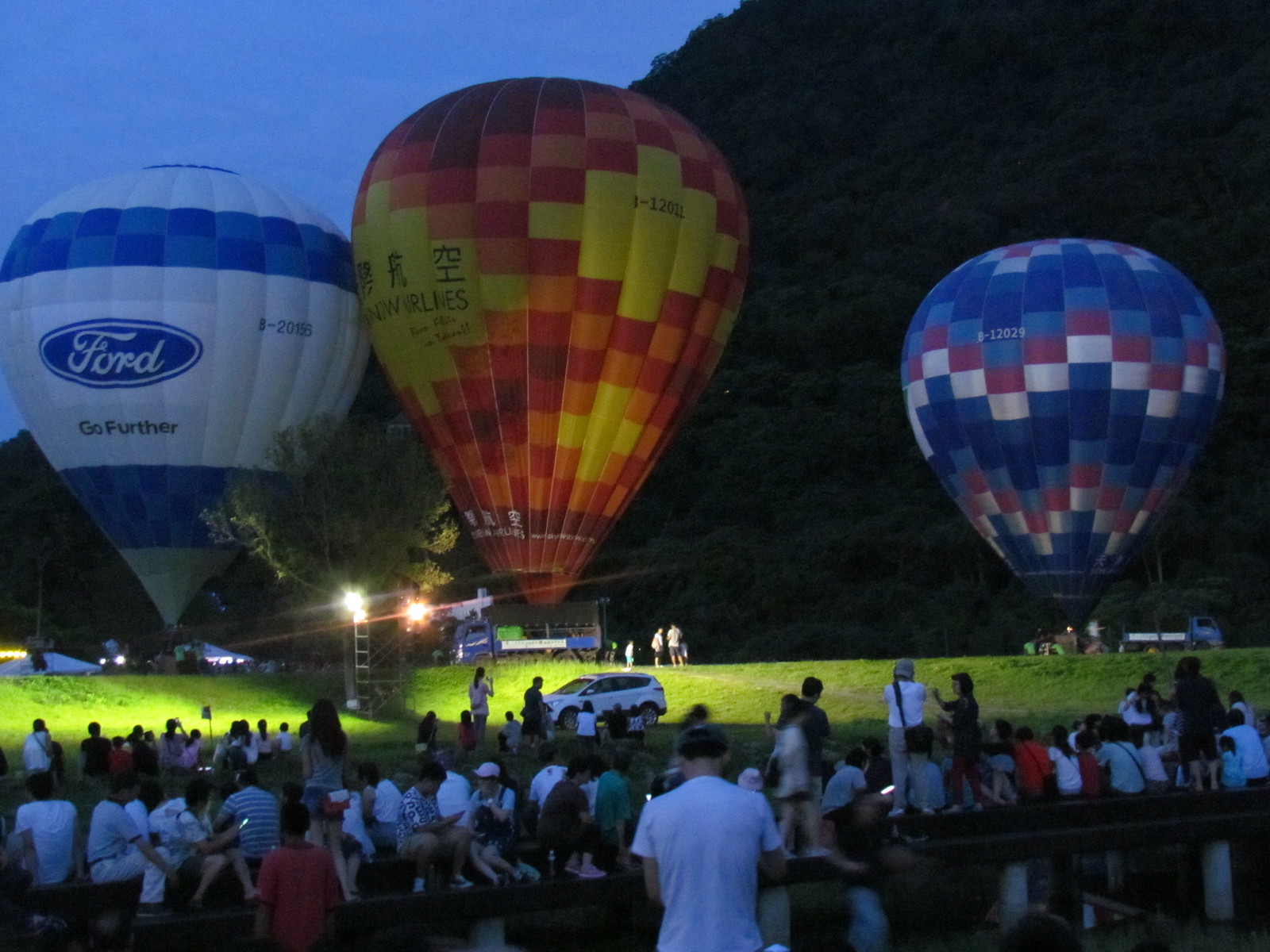This color photograph depicts a serene yet vibrant scene of three hot air balloons preparing for liftoff in an open field at dusk. The setting is adorned with soft lights as a large crowd clad in summer attire gathers to witness this annual event. In the foreground, a mixture of over a hundred people, standing and sitting, creates an animated yet harmonious atmosphere. On the right side of the image, a towering mountain looms, its dark silhouette contrasting with the gradually brightening sky. 

The three hot air balloons, tethered to truck beds, stand majestically on the field. On the far left is a white balloon adorned with blue stripes and the Ford emblem, accompanied by the slogan "Go Further." In the center, the largest balloon bursts with vibrant hues of yellow, orange, and red and features intricate designs with some Chinese characters, although their meaning remains unclear. On the far right, a smaller balloon showcases a pattern in shades of blue, red, and white, and bears the number B-12029. A single tree can be seen between the second and third balloons, contributing to the picturesque setting, while a solitary white car is parked among the crowd, further emphasizing the communal nature of this charming event.